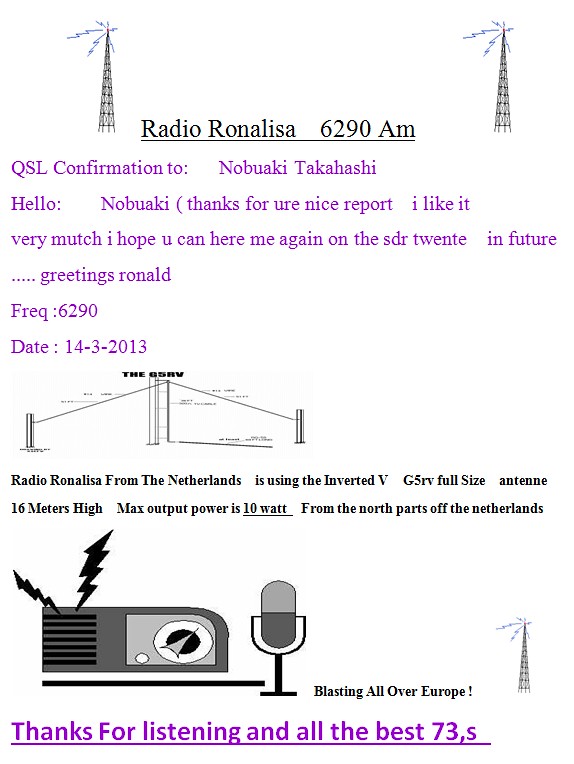The image, primarily text-based with several black-and-white illustrations, appears to be a QSL confirmation for a radio station called Radio Ronalisa, broadcasting at 6290 AM. At the top center, flanked by two black radio towers emitting blue lightning-like streaks, is the title "Radio Ronalisa 6290 AM" in underlined black text. Below this, in purple text, is a personalized message: "QSL Confirmation to Nobuaki Takahashi. Hello Nobuaki, thanks for your nice report. I like it very much. I hope you can hear me again on SDR 20 in the future... greetings Ronald." Following this, the frequency "6290" and the date "14-3-2013" are listed. 

The document provides technical details about the station, stating: "Radio Ronalisa from the Netherlands is using an Inverted G5RV full-size antenna, 16 meters high, with a maximum output power of 10 watts from the northern parts of the Netherlands, blasting all over Europe." 

An illustration at the bottom features a vintage-style radio with sparks emanating from its speakers, signifying sound or broadcast waves. To the right of the radio is a detailed drawing of a microphone on a stand, with the microphone itself described as pill-shaped, having a light gray top and dark gray bottom. Further to the right is another radio tower illustration with electric bolts emerging from it.

The message concludes in purple text: "Thanks for listening. All the best. 73S." This caption is set against a white background.